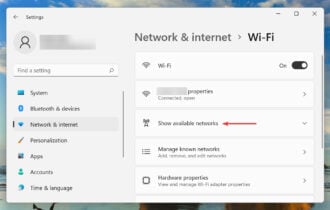A user interface view captured on a laptop screen displaying the Network and Internet settings, specifically the Wi-Fi settings. The rectangular screen is oriented horizontally with the desktop background featuring a serene seascape with clouds. The settings window occupies the majority of the screen, divided into a two-section layout.

On the left side, a vertical menu lists various system settings categories, including System, Bluetooth & Devices, Network & Internet, Personalization, Apps, Accounts, Time & Language, and more. Some of the text in the menu is partially illegible, likely due to the small screen size and resolution.

In the main section to the right, the focus is on Network & Internet settings, with a particular emphasis on Wi-Fi options. Wi-Fi is toggled on, and several subsections are available, possibly indicated by right-facing arrows and collapsible menus. These options likely include:
- Show available networks
- Manage known networks
- Properties
- A potential feature for sharing network settings or properties (the text is unclear).

Additionally, the settings window features standard window controls: a left-facing arrow for navigation, an 'X' for closing the window, and a dash (-) for minimizing it. At the top-right corner of the window, a user profile icon resembling the upper body of a snowman within a circle suggests that user-specific settings might be available.

This screenshot provides a detailed view of the Network & Internet settings interface, designed for adjusting Wi-Fi connectivity and other related preferences on the laptop.